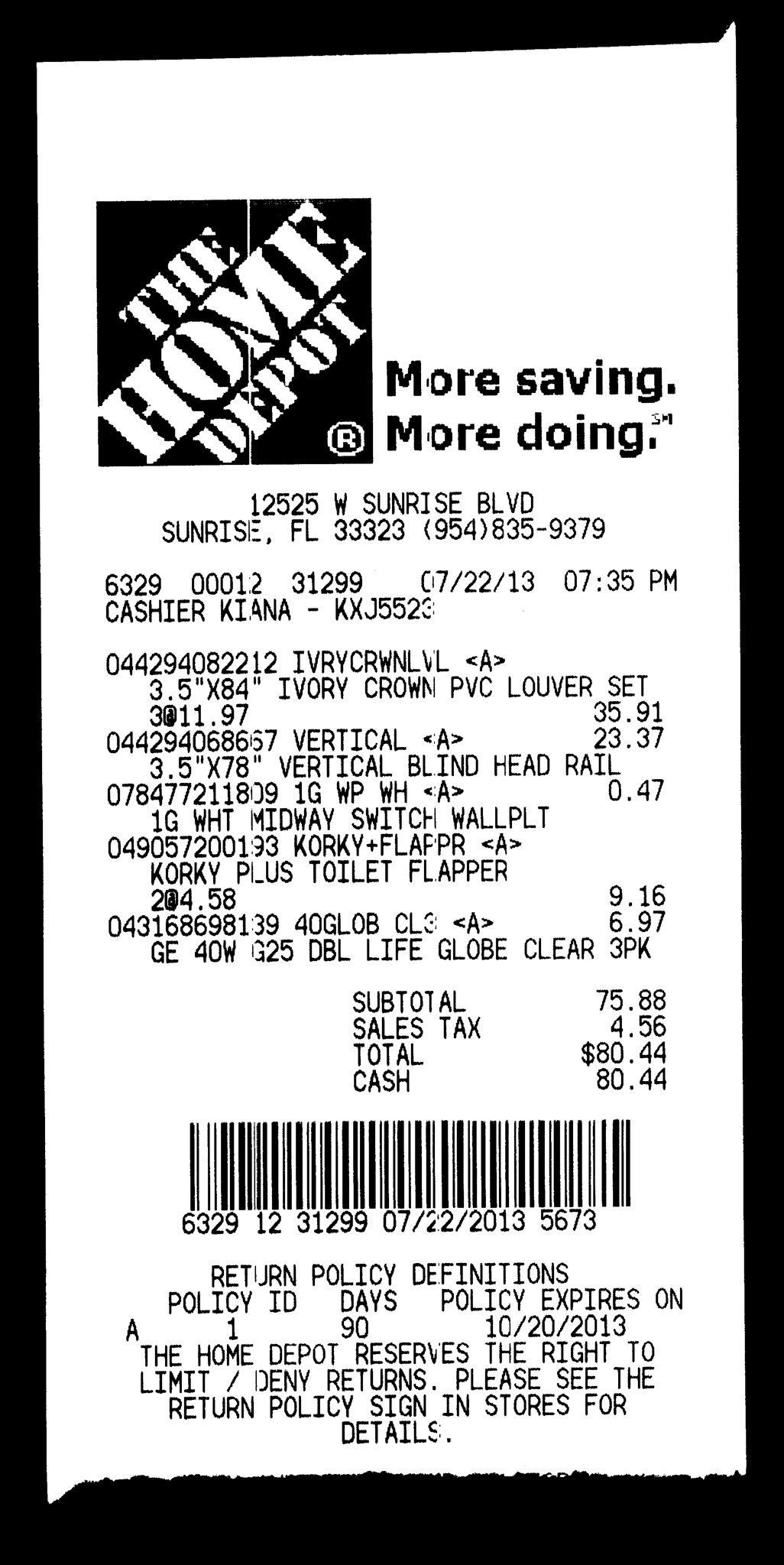A detailed caption of the image would be:

"The image features a white till receipt from The Home Depot, prominently displayed against a stark black background. The receipt details a variety of purchased items such as wallpaper, vertical blinds, louvers, and a toilet flapper. The store's slogan, 'More Saving. More Doing.', is clearly visible, reinforcing its branding message. The total amount paid in cash is $80.44. At the bottom of the receipt, a barcode is present, accompanied by The Home Depot's return policy, which states: 'The Home Depot reserves the right to limit or deny returns. Please see the return policy sign in stores for details.' This message highlights the store’s strict return guidelines."